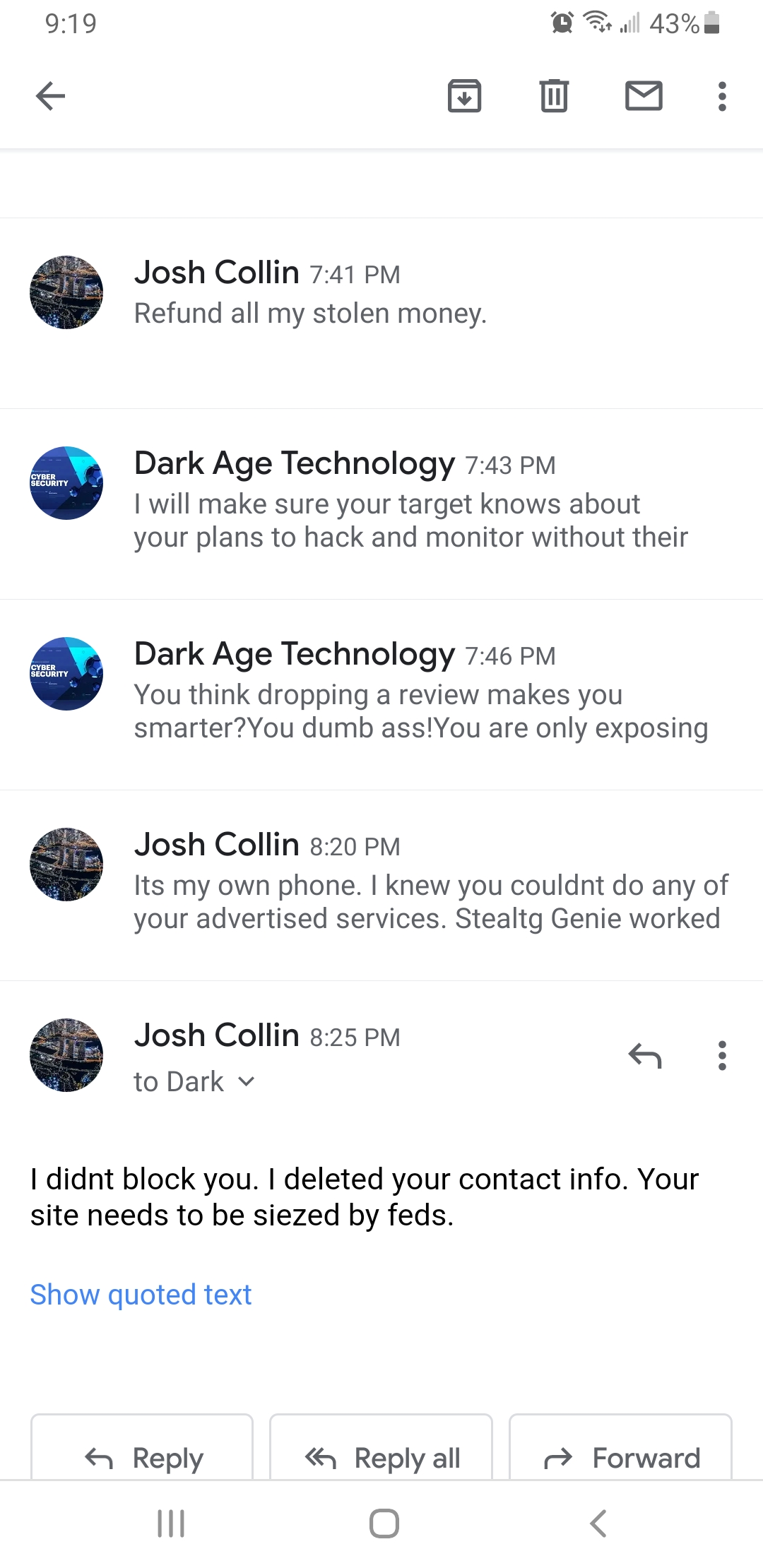**Detailed Caption:**

The image captures a heated conversation between Josh Collin and DarkAge Technology within an email interface. At the very top of the screen, there's an arrow pointing to the left, indicating a back navigation option. Above this arrow, the time is displayed as 9:19, accompanied by an alarm bell icon to its right, a Wi-Fi signal icon with two bars lit, and a battery icon showing 43% charge.

Below the time and status icons, there is a navigation bar with another left-pointing arrow, followed by four icons: a down arrow within a box, a trash can, an envelope, and three vertical ellipses. These icons are likely for downloading the email, deleting it, marking it as unread, and accessing more options, respectively.

A light gray line demarcates these navigation elements from the conversation below. The conversation, set against a white background, begins with visible avatars for each participant, though the details of these avatars are unclear.

- **Josh Collin** at 7:41 PM: "Refund all my stolen money."
- **DarkAge Technology** at 7:43 PM: "I will make sure your target knows about your plans to hack and monitor what's out there and it doesn't say anything else."

Each message is separated by a faint horizontal line. The interaction continues:

- **DarkAge Technology** at 7:46 PM: "You think dropping a review makes you smarter? You dumbass, you're only exposing."
- **Josh Collin** at 8:20 PM: "It's my own phone. I knew you couldn't do any of your advertised services. STEALTG, it should be H. I think it's meant to be Silph Genie worked."
- **Josh Collin** at 8:25 PM: "I didn't block you. I deleted your contact info. Your site needs to be seized by feds."

Josh Collin’s last response is highlighted with another left-pointing arrow and three vertical ellipses, also featuring a blue link labeled "show quoted text."

At the bottom of the email interface, three buttons are embedded within light gray boxes: "Reply" (left arrow), "Reply All" (left arrow with an additional arrowhead), and "Forward" (right arrow with the word "Forward"). These buttons have a white background with dark gray or black text.

Finally, at the very bottom, there are icons for three vertical lines, a semi-square with rounded edges, and a left-pointing arrowhead or less-than sign.